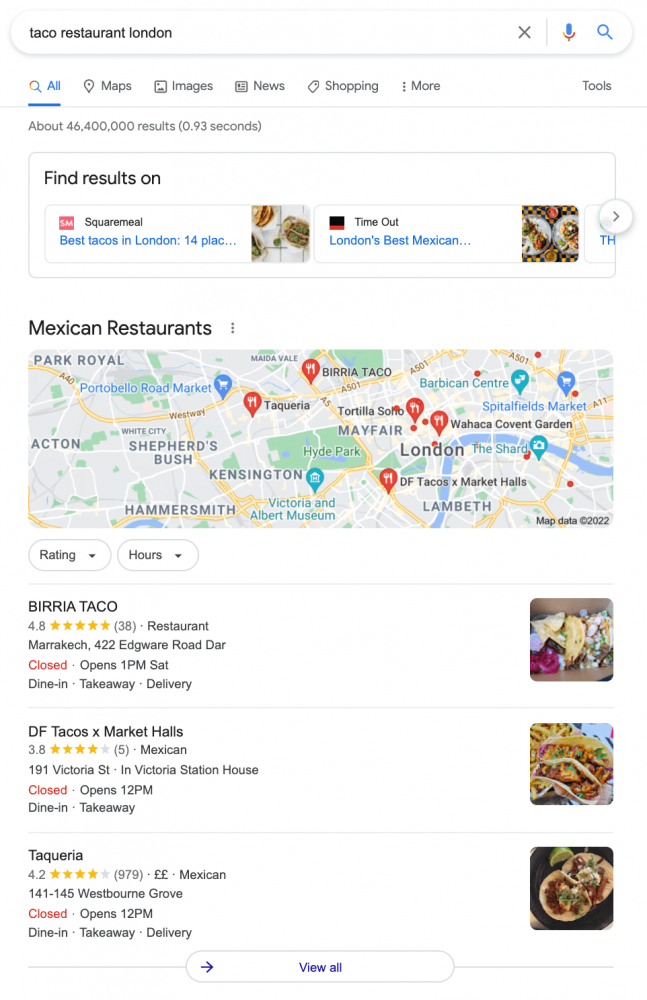This image captures a Google search result for a taco restaurant in London using the traditional Google Chrome interface. Below the search bar, the "All" category is selected, with options to switch to "Maps," "Images," "News," "Shopping," and more for refined results. An advertisement is prominently displayed beneath these tabs, offering additional clickable results in a designated ad box.

Further down, the search results include a section labeled "Mexican restaurants," featuring a map of London marked with red indicators to highlight the locations of several taco restaurants. The map shows three specific venues: Burrito Taco, DF Tacos, and Taqueria. Each restaurant is accompanied by an image, presumably uploaded by users, depicting food or the establishment itself.

Details about the restaurants reveal their current status and ratings. All three are indicated as being closed at the time of the search. Burrito Taco boasts a high rating of 4.8 out of 5, DF Tacos holds a lower rating of 3.8, and Taqueria has a respectable rating of 4.2.